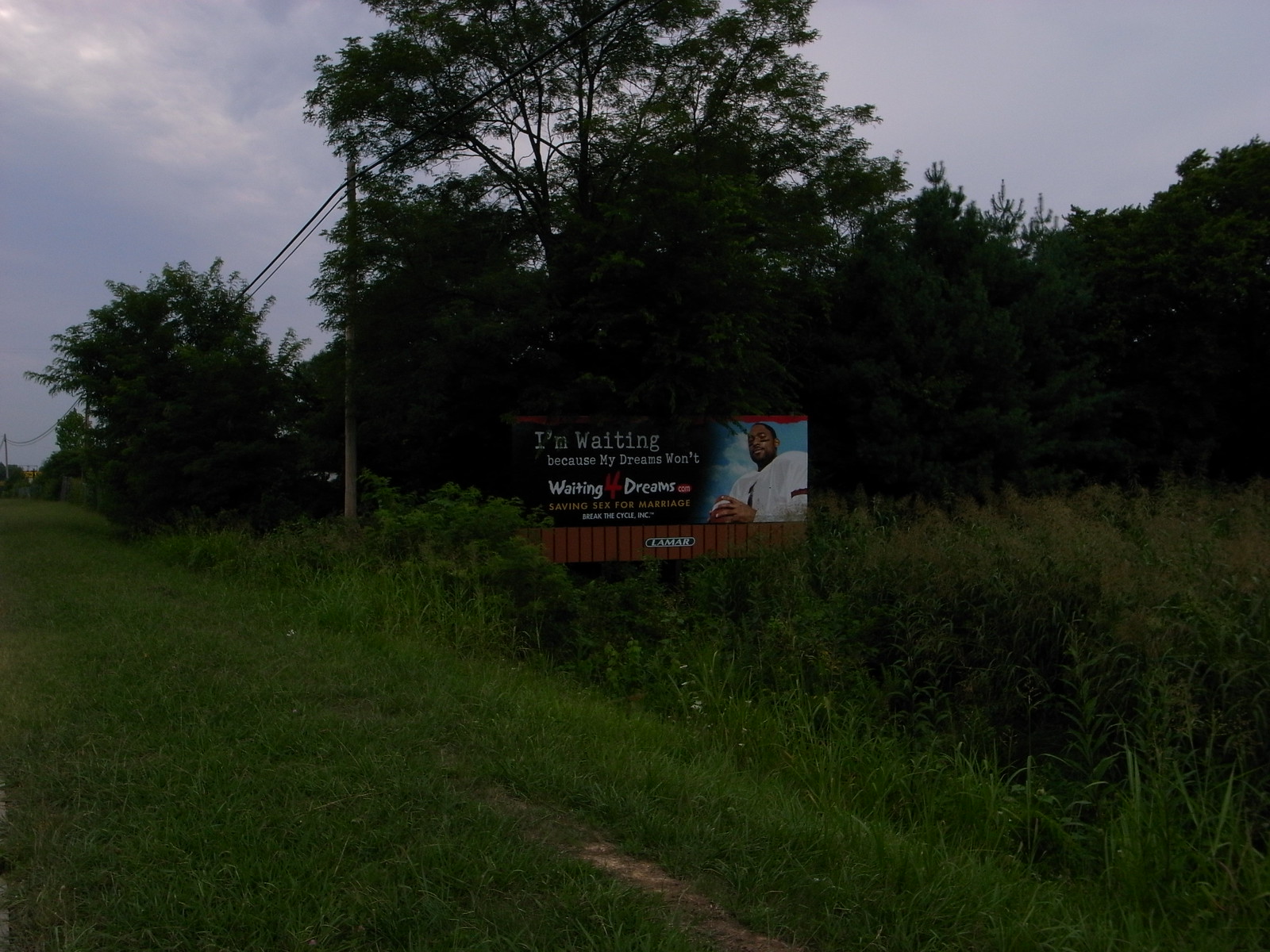The image depicts a dark, outdoor scene of an overgrown field characterized by green grass and reddish dirt. In the background, taller grasses and numerous trees frame an advertising billboard. The billboard, partially obscured by the foliage, displays white text on a black background, with the message: "I am waiting because my dreams won't" and "waiting for dreams," using a red number four to represent the word "for." An additional phrase, possibly ".com," appears in white with red edging, along with the phrase "saving sex for marriage."

The central figure on the billboard is an African man wearing what looks like a white football jersey, highlighted by black swatches under his eyes, and sporting short hair and a beard. Above him, a cloudy sky with limited blue hue blends into the scene. A telephone pole and wires are noticeable, hinting at a rural setting. The surroundings are lush with various bushes, weeds, and shrubs, invoking the atmosphere of a countryside or farmland area, potentially along an old dirt track or walking path.